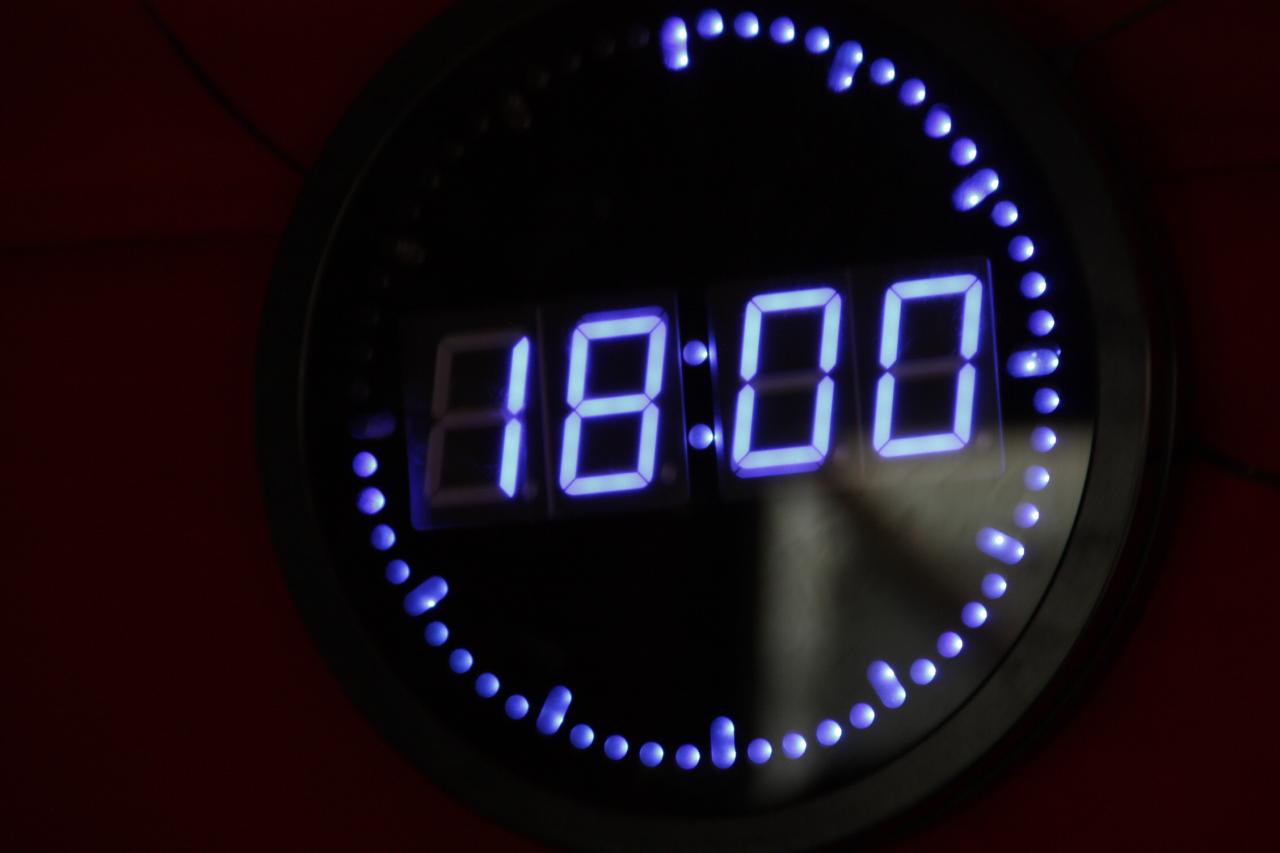In this rectangular image, a black background accentuates a wall clock featuring a digital display. The clock displays the time "18:00" in a bluish-white, illuminated digital font. Surrounding the digital display is a faint circular outline, suggesting the classic shape of a wall clock. Notably, the top quarter of the clock's outline is dark and unlit. The rest of the clock face is adorned with small circular dots and lines marking each hour and every 15-minute interval. The solid black background is subtly brightened by a slight reflection from the digital lights, particularly illuminating the lower right section of the image.